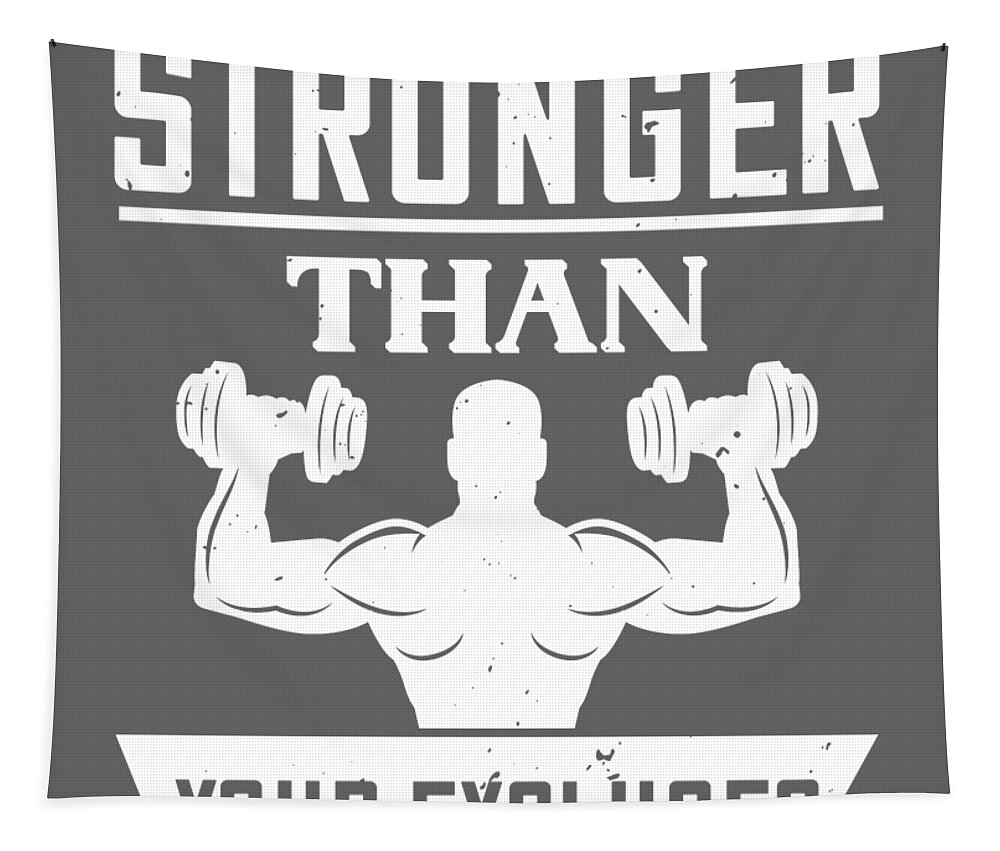The image features a central banner with a medium gray background situated on a larger white canvas. At the top of the banner, bold white text reads "STRONGER THAN," with a horizontal line beneath "STRONGER." The centerpiece is an illustration of the back of a bald, muscular bodybuilder, depicted in silhouette style, emphasizing his well-defined muscles. He is seen performing an overhead press with two dumbbells, each with four plates of varying sizes. The lower part of the banner has a white section with an undisclosed text that is partially cut off, preventing it from being fully read. The banner gives an impression of either a sign or a graphic, possibly used for inspirational purposes.